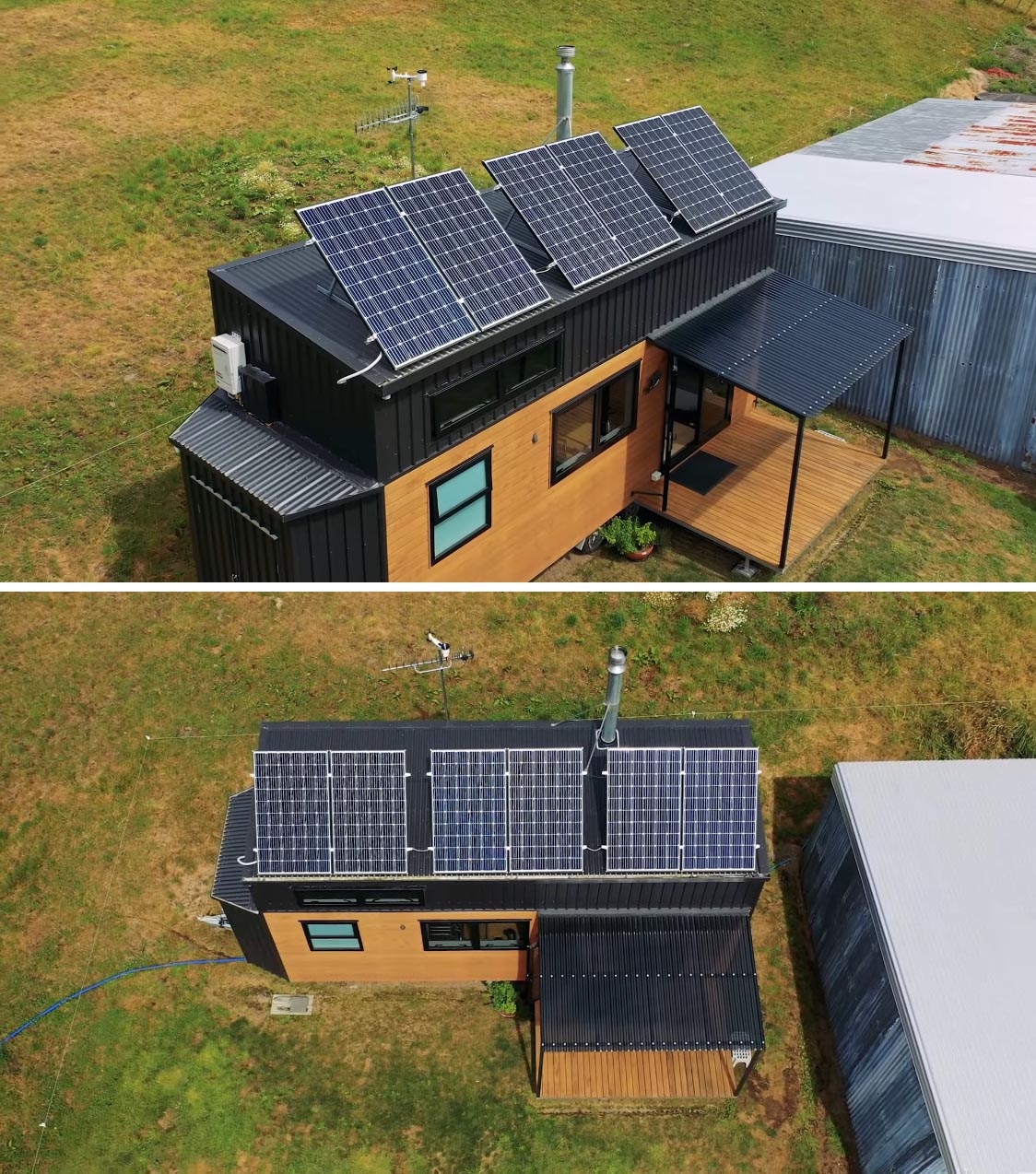The image features an outdoor, daytime scene with bright lighting, though the sky is not visible. A well-built tiny home stands as the centerpiece, constructed with a combination of dark gray and brownish wood siding. The front wall of the house has two windows—one with shades and one without. The entrance is a glass sliding door, accompanied by a black mat. 

The porch, featuring wooden flooring, is covered by a roof made from a black material. The house itself is equipped with three large solar panels affixed to its black roof, denoting an effort to harness solar energy. An additional solar panel can be seen on the deck area of the house.

The upper half of the house also includes a window framed by black siding. The home is situated in a spacious green yard with touches of yellow in the grass, next to a barn or similar structure possibly made of metal or zinc. The detailed view highlights the home's modern, energy-efficient design amidst a serene, verdant environment.